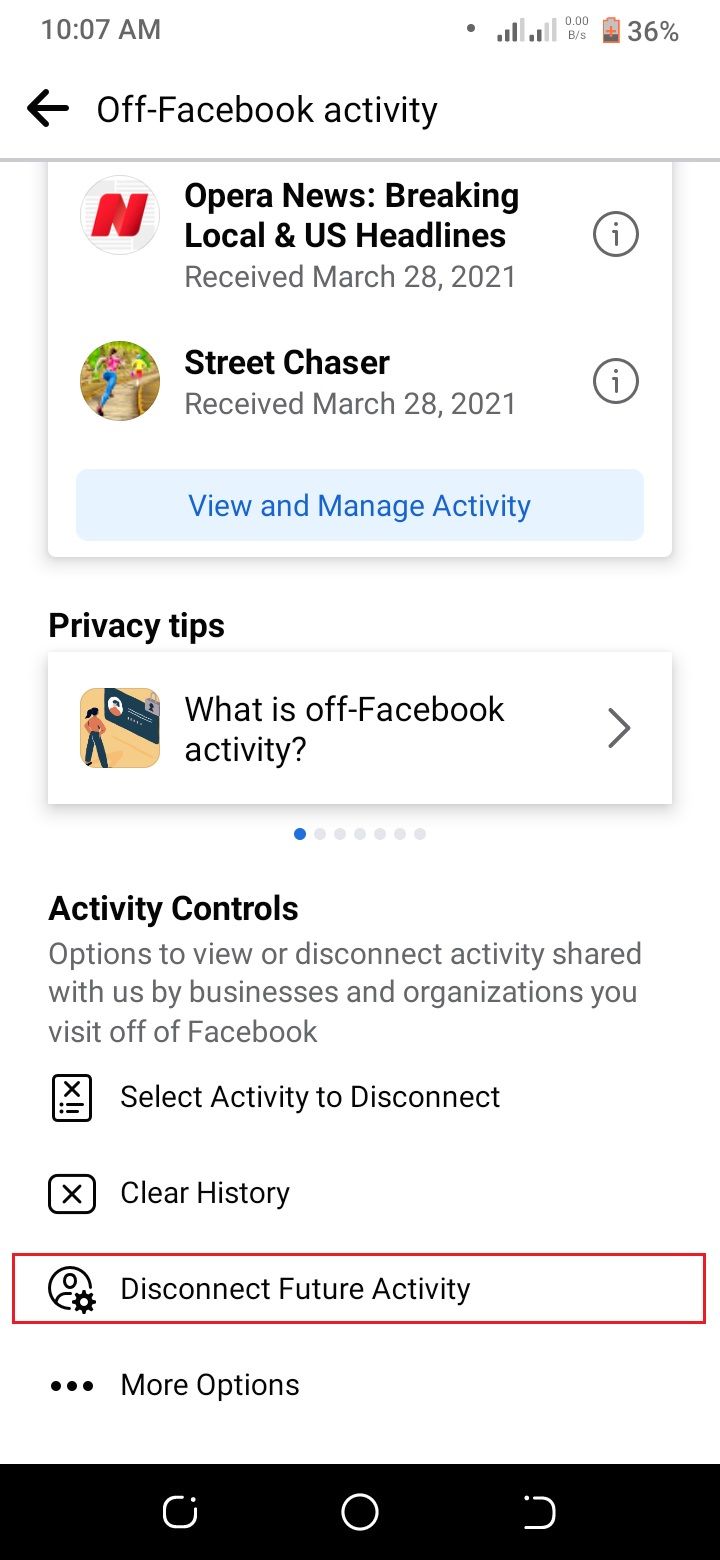A detailed screenshot from a cell phone showing a menu with a white background. At the top of the screen, the phone's status bar is visible, indicating the time as 10:07 AM on the left and displaying the connection status on the right. The battery level is at 36%, with the battery indicator highlighted in red, signifying a low charge.

Beneath the status bar, a bold, dark black left-pointing arrow is labeled "Off Facebook Activity." Below this heading, several categories are listed: "News," "Privacy Tips," and "Activity Controls."

In the section labeled "Activity Controls," there is a black horizontal rectangle with a circular button in the center. To the left of this is a rounded rectangle icon, and to the right, highlighted in a red box, is an option labeled "Disconnect Future Activity." Above this is a section titled "Clear History, Select Activity, Disconnect."

In the news section, it lists "Opera News, Breaking Local and U.S. Headlines" alongside a gray circle with an information eye icon. Below this, it mentions "Street Chaser, Received March 28, 2021," with the same information icon next to it. Finally, there is a blue clickable link labeled "View and Manage Activity."